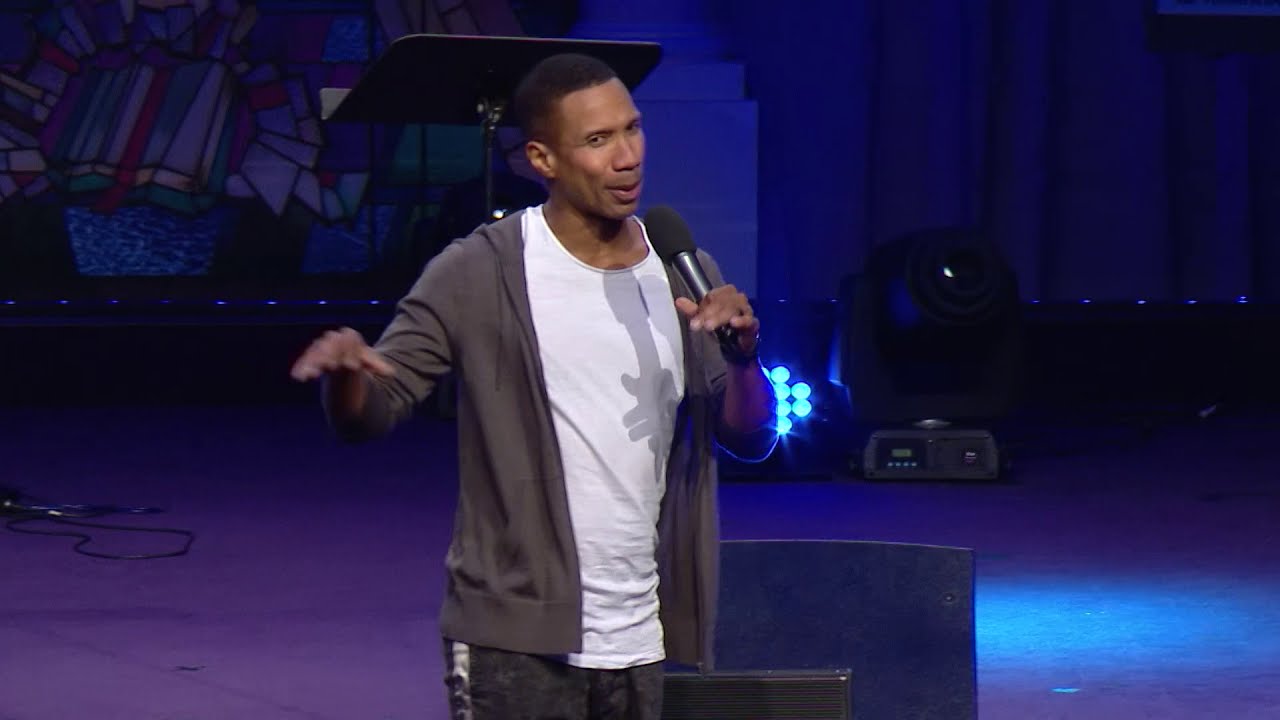In this vibrant photograph, a black man with short black hair is captured on a dimly lit stage, speaking animatedly into a microphone held in his left hand. His right hand is outstretched, fingers open at chest level, adding emphasis to his speech. He wears a white shirt beneath a charcoal gray sweater that reaches just below his elbows, paired with black pants featuring a distinct silver stripe on the left pant leg. The background is dramatically dark, illuminated by striking light blue spotlights, casting a shadow of the microphone onto his chest and creating a visually dynamic scene. There’s a podium stand positioned above his head, hinting at a formal engagement, and a stained glass or painted window adds a splash of color to the backdrop. The setting suggests he may be a comedian delivering a punchline or a preacher sharing a message, deeply engaged with his unseen audience.